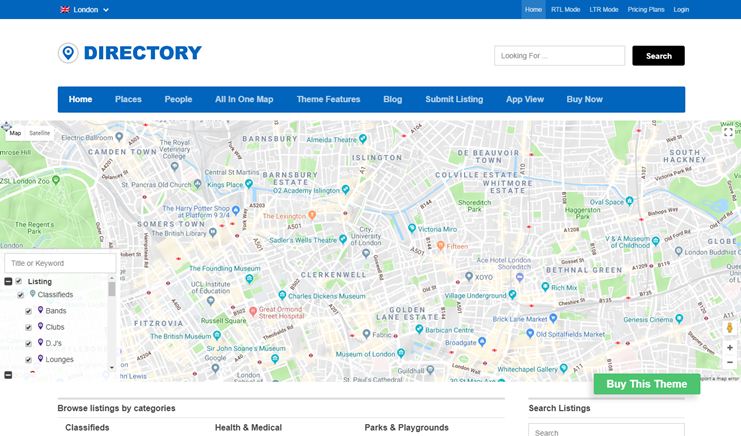Screenshot of a Website:

At the top of the screenshot, a blue bar spans the width of the website. On the left side of this bar, a red shopping cart icon is situated next to the word "London" in bold white font, accompanied by a small white downward arrow. To the right of these elements, several menu options are listed in white font: "Home" (which is currently selected), "RTL Mode," "LTR Mode," "Pricing Plans," and "Login."

Directly beneath the blue bar, a white rectangle hosts various elements. In the upper left corner of the rectangle is a blue circle with a location-sharing symbol inside it, followed by the word "Directory" in bold blue font. Adjacent to this, a white search field with placeholder text in grey font reading "Looking for..." is positioned. Next to the search field is a black button labeled "Search" in white font.

Below the white rectangle, a blue navigation bar lists additional options in white font: "Home," "Places," "People," "All-In-One Map," "Theme Features," "Blog," "Submit Listing," "App View," and "Buy Now."

The primary content of the page features a detailed graphic of a street map, likely of London, given the context provided. The map displays numerous streets and landmarks, all clearly labeled. Various points of interest are indicated by little blue arrows scattered throughout the map, highlighting notable locations.